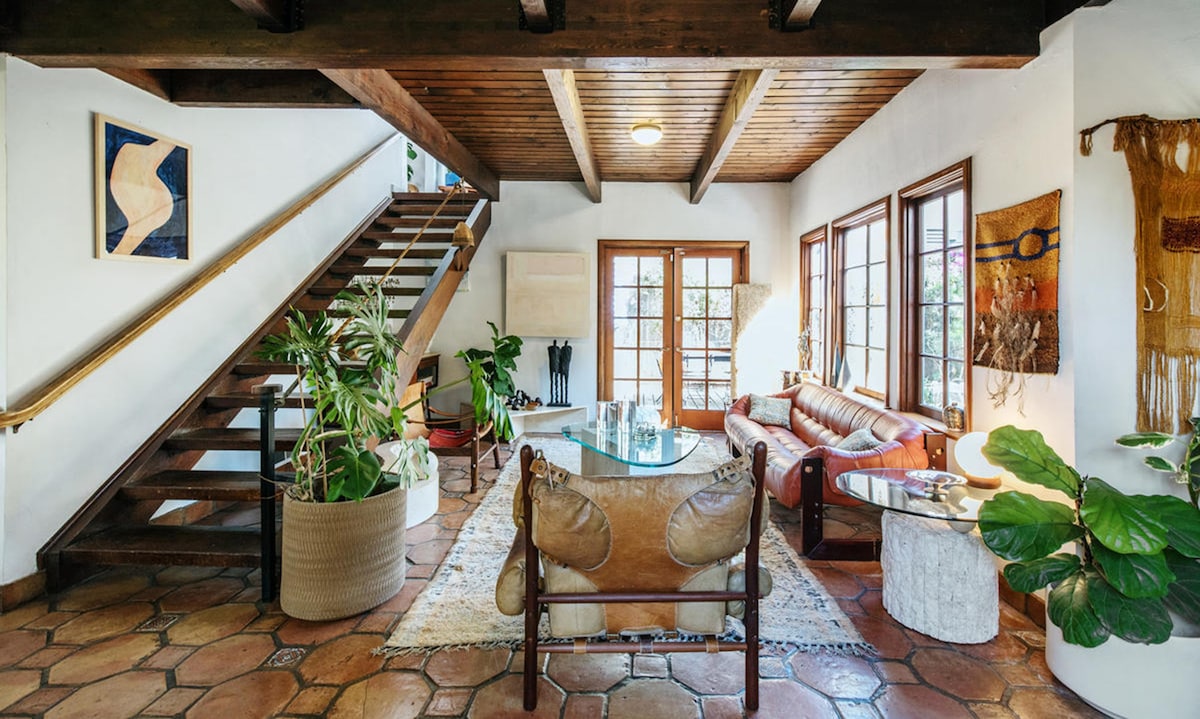This detailed image depicts a cozy living room with a distinct Bohemian aesthetic. Dominated by shades of brown, beige, and cream, the space features a prominent wooden staircase equipped with a light beige handrail, that leads to the next floor. Below the staircase, a green plant in a beige planter adds a touch of natural color. The room’s ceiling is brown with a round, yellow light fixture hanging from it.

The walls are primarily white, with the far-left wall displaying a curious portrait or artwork resembling white and peach hues, accented by blue. Across the room, a brown leather sofa sits against a wall adorned with three brown-framed windows with glass inserts, filling the space with natural light. Adjacent to the sofa, another piece of artwork—described as blankets with long cloth strands—adds to the room’s eclectic charm. 

A glass table is situated on the far right, near an additional green plant. The floor is covered in hexagon-shaped tiles, adding texture and complexity to the room's design. Each element, from the wooden door with glass inserts to the mix of small plant pots, chairs, and sofas, contributes to the overall warm, inviting ambiance of the living area.